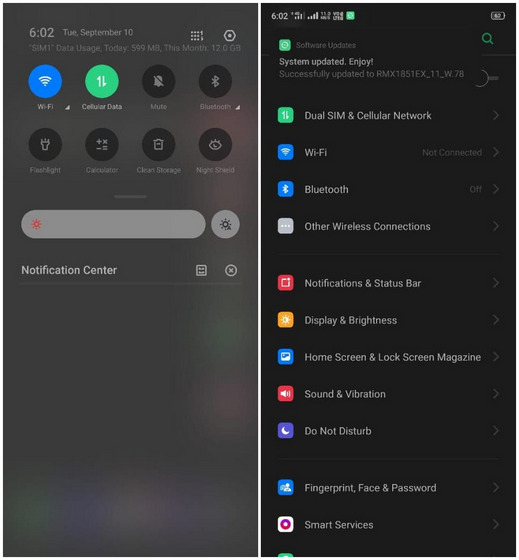The image consists of two side-by-side screenshots from an Android mobile device, both displayed in dark mode.

The left screenshot showcases the device's notification center and quick settings panel, which occupies the entire screen. The lower half of the screenshot displays an empty notification center, indicating no notifications at present. The upper half features the quick settings area. It shows the current time as 6:02 on Tuesday, September 10th. The Wi-Fi icon is illuminated in blue, signifying it is enabled, and the cellular data icon is illuminated in green. Several other quick setting icons are visible but not activated, including mute, Bluetooth, flashlight, calculator, clean storage, and night shield. The brightness level slider is also present, though its precise position is unclear as it appears solid.

The right screenshot reveals the settings menu of the device, set against a dark background. This menu lists various settings options with colorful icons beside each: Wi-Fi, Bluetooth, notifications, status bar, display and brightness, home and lock screen magazine, do not disturb, fingerprint, face and password. Each icon is distinctively colored in hues such as green, yellow, blue, purple, and red, providing visual differentiation between the categories.